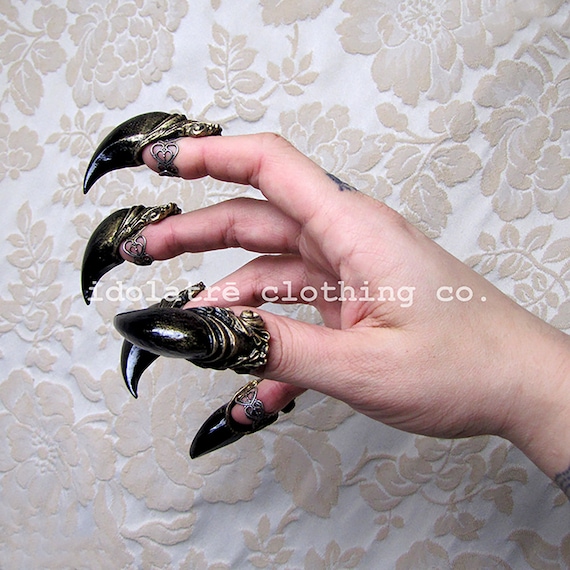A close-up image depicts a woman's hand adorned with elaborate, claw-like nail pieces that resemble jewelry. These unique accessories have a silver metallic base that fits over the fingers, extending into large, spiky, black talons that are sharply pointed and shiny. The hand, appearing to belong to a light-skinned woman, is held out against a fabric background with a beige floral pattern. The fabric shows various intricate leaves and flower petals, creating a lush botanical backdrop. Additionally, there is a visible watermark on the fabric that reads "Idolatry Clothing Co." in white letters. The hand also features a tattoo on the pointer finger and another on the wrist, adding to the overall ornate appearance of the image.